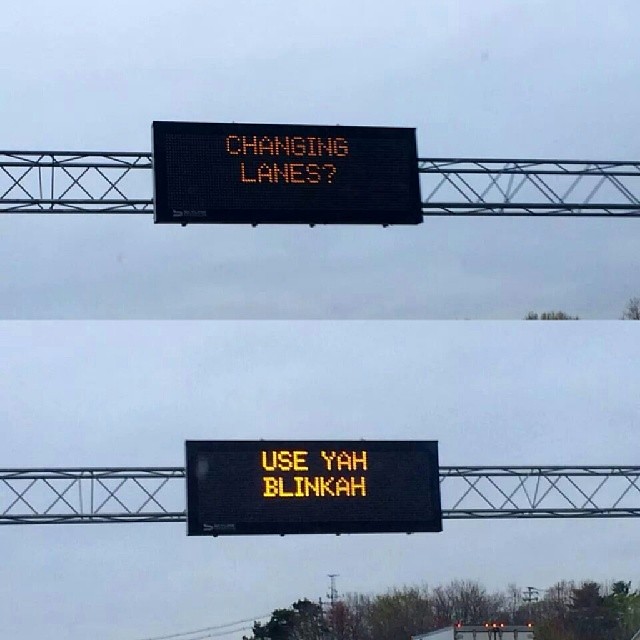This outdoor color photograph depicts a split image featuring two separate shots of the same electronic street sign taken from a slowly approaching vehicle. Both images show a large rectangular black digital sign supported by metal latticework on either side. In the top half, the sign displays the message "Changing lanes?" in bright orange text against a hazy light blue sky. The lower half features the same sign displaying "Use ya blinkah" in yellow text, with additional elements such as trees, the roof of a tractor-trailer, and its trailing lights visible in the background. The upper image appears slightly darker than the lower one, suggesting different weather conditions and lighting at the times the photos were taken.